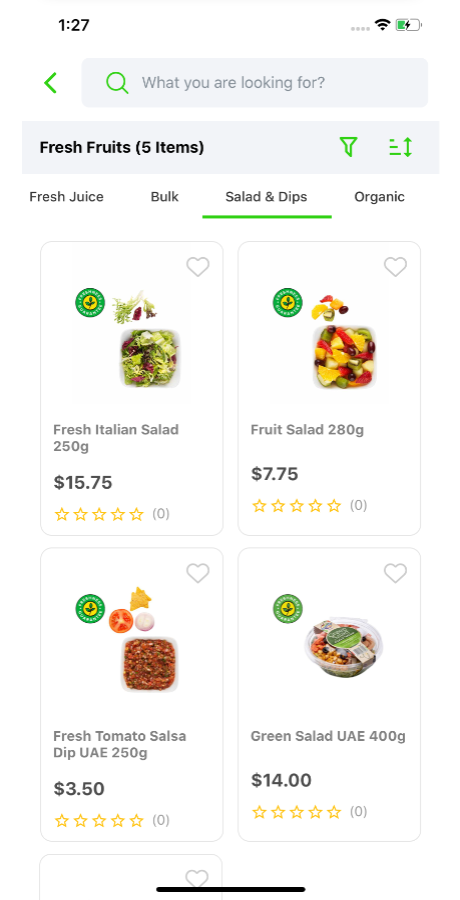The image showcases a search interface where the search bar is currently empty. The highlighted category is "Fresh Fruits" with a total of five items listed. Below this, there are options to browse other categories such as "Fresh Juice," "Bulk," "Salads and Dips," and "Organic."

Within the "Salads and Dips" category, four items are displayed in a grid format, two across and two down. The top left item is "Fresh Italian Salad," weighing 250 grams and priced at $15.75. To its right is "Fruit Salad," weighing 280 grams and priced at $7.75. In the bottom left is "Fresh Tomato Salsa Dip" from the UAE, weighing 250 grams and priced at $3.50. Next to it, on the bottom right, is "Green Salad" also from the UAE, weighing 400 grams and priced at $14. Each item features a five-star rating option, though none have been clicked, and there are zero reviews for all products.